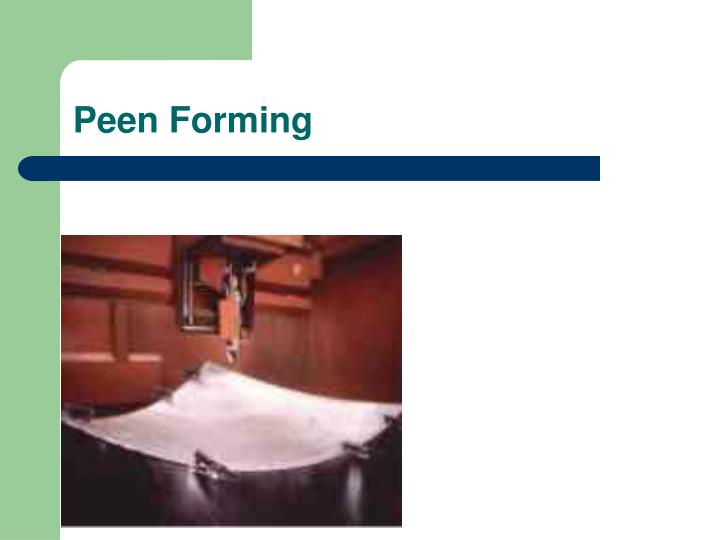This image, likely from a PowerPoint presentation or pamphlet, features a detailed layout with the title "Peen Forming" prominently displayed at the top. Set against a white background, a pale green bracket curves around the top left corner, complemented by a horizontal thick dark blue line directly below the title. This blue line has a rounded end on the left and a straight end on the right, adding a structured visual element. 

Beneath this, the central photograph depicts a large piece of machinery designed to hammer down onto a metal sheet. The metal sheet is positioned on a black table, secured in place by straps or clips along its edges. The machine appears active, with the press poised to strike repeatedly. Surrounding the machinery, there is a clear white space, and the machine is set against a backdrop of medium-colored wooden paneling, which provides a neutral yet contrasting background to the industrial scene in the foreground.